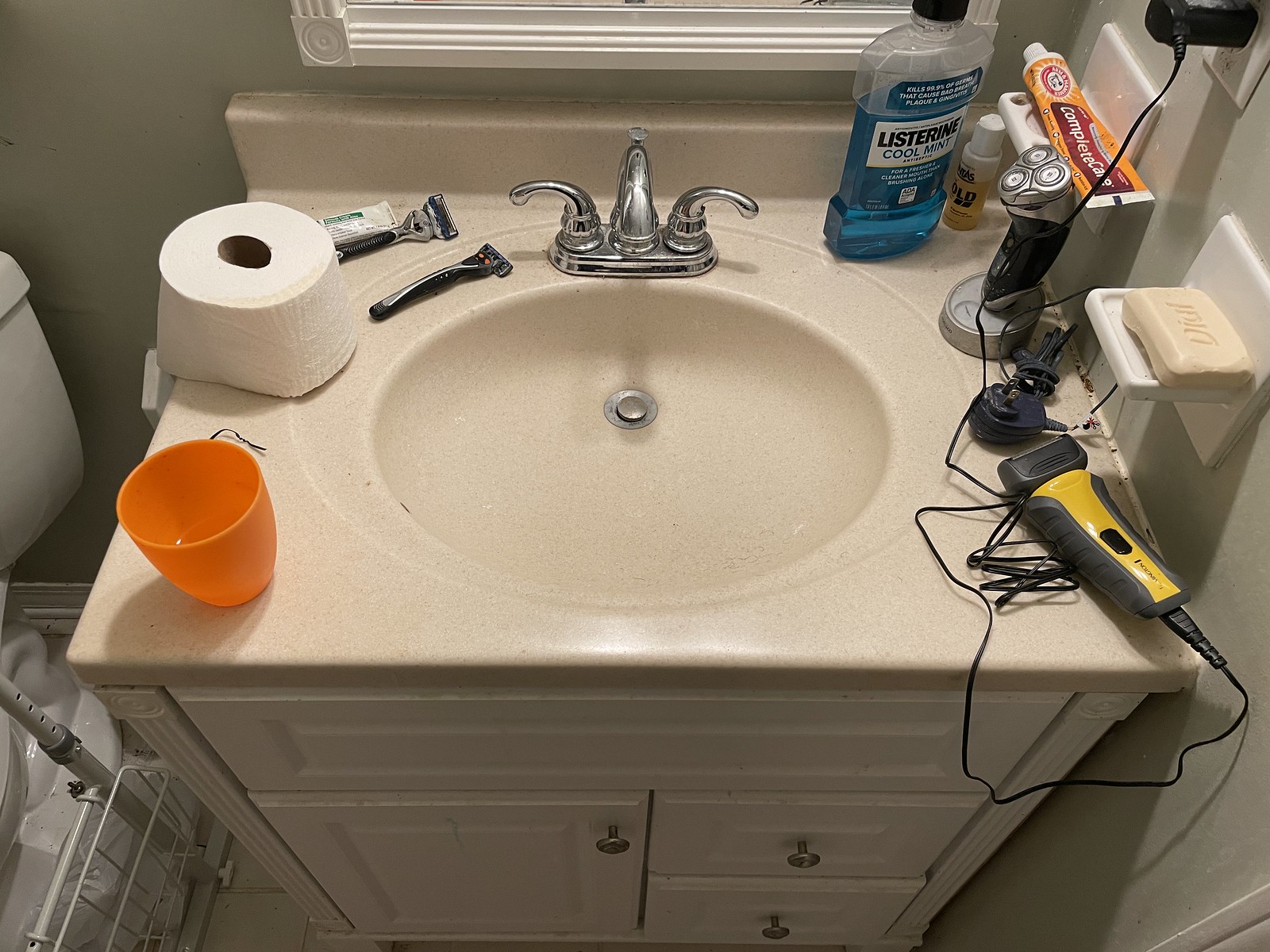The close-up image highlights a beige bathroom sink and countertop with matching beige cabinets and drawers below. To the left of the sink, a roll of white toilet paper is placed alongside an orange plastic cup and two shaving razors. On the right side, a clear bottle of blue Listerine mouthwash with a black cap stands next to a tube of Arm & Hammer toothpaste in yellow and red packaging, labeled "Complete Care." Additionally, an electric shaver and a yellow and black barber's clip, plugged into an electrical outlet, appear on the countertop.